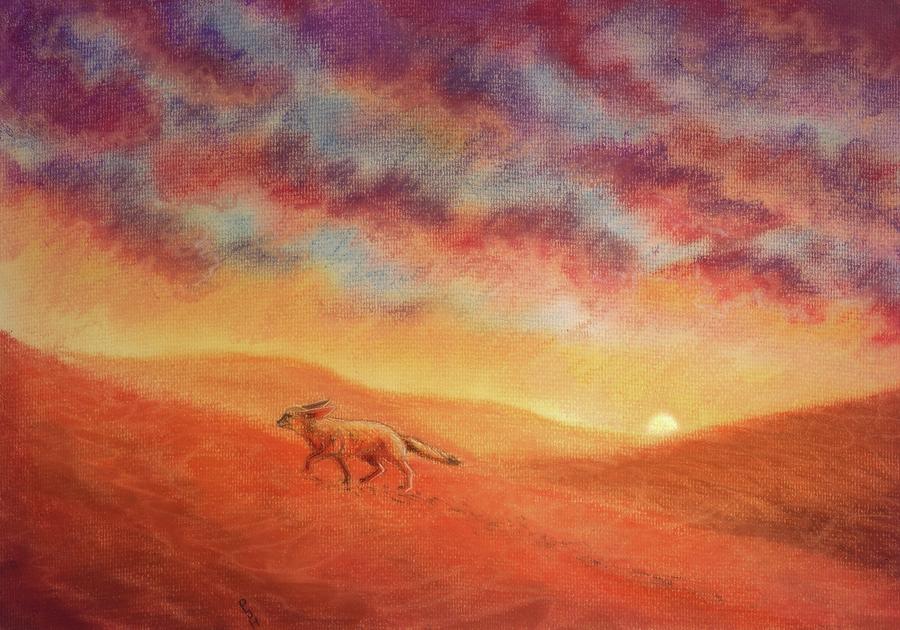The image appears to be an AI-generated or hand-drawn illustration rather than a realistic photo. It features a single animal, which resembles a wolf, though it could also be interpreted as a fox. Positioned in the bottom center, the creature is depicted running or walking up what appears to be a sandy hill or dune. The animal's tail is down, and its right paw is placed slightly forward of its left, giving a sense of motion. Its ears are pointed backwards, possibly indicating alertness or focus on its path.

In the background, the sky exhibits a stunning gradient of colors—purple, red, and blue blending into pinks as they meet the horizon. Near the setting sun, which is white and peeks through some planes, these colors transition into warm hues of yellow and orange. The scenery behind the animal depicts hills or mountains, their colors becoming darker and more orange towards the front of the image. The rich, varied palette also includes browns and a melanin range, contributing to the overall vibrant and dynamic atmosphere of the scene. The composition is devoid of any other animals or text, emphasizing the solitary journey of the central figure against the backdrop of a spectacular sunset.